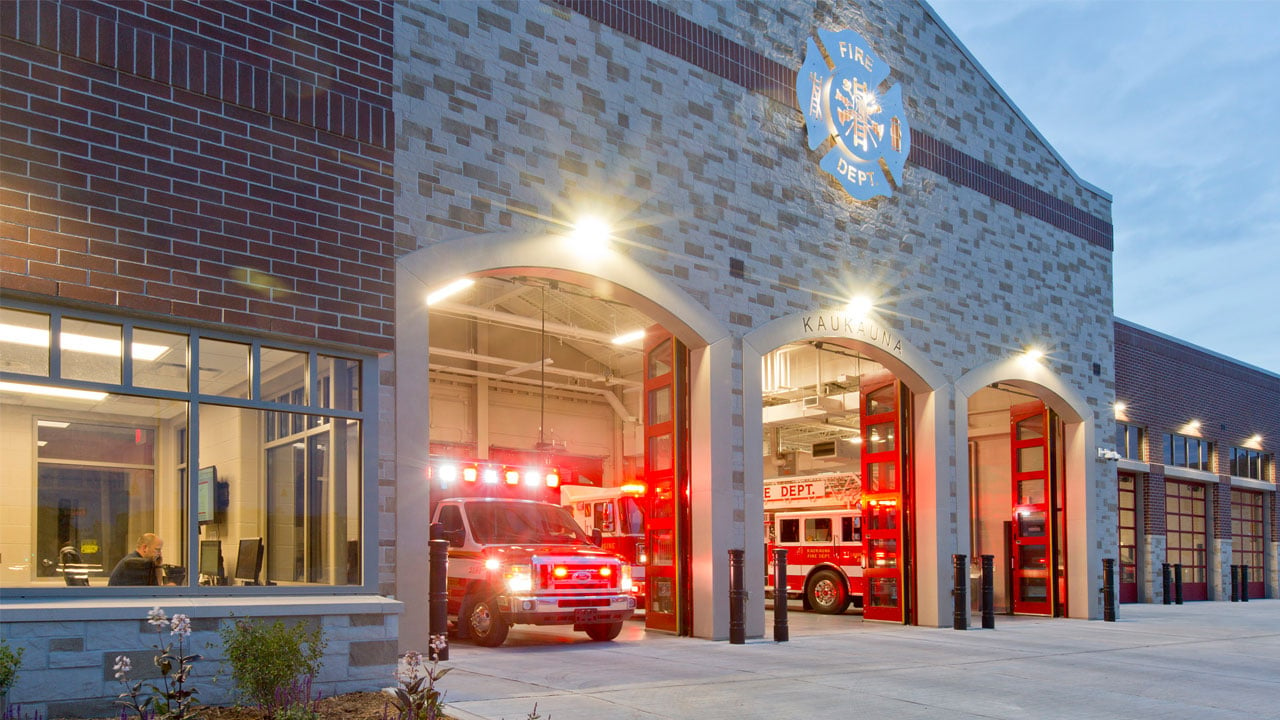The image depicts a well-maintained fire station with a tall, handsome facade. Prominently, there is a large roundish sign near the roofline that reads "Fire Department" in gold letters against a blue background, accompanied by a flower-shaped logo with four blue petals. Below, three arched entries lead into the firehouse, each with red doors wide open, revealing emergency vehicles inside. The central arch has additional text above it spelling "cacaona."

Inside the garage area, three emergency vehicles are visible. The central vehicle appears to be a fire truck with a folded ladder, marked as "DEPT." To the left is another emergency vehicle, while on the far left is a pickup truck. On the left side of the building, through the windows of a small office, a man can be seen at a desk, looking at a computer and possibly talking on the phone.